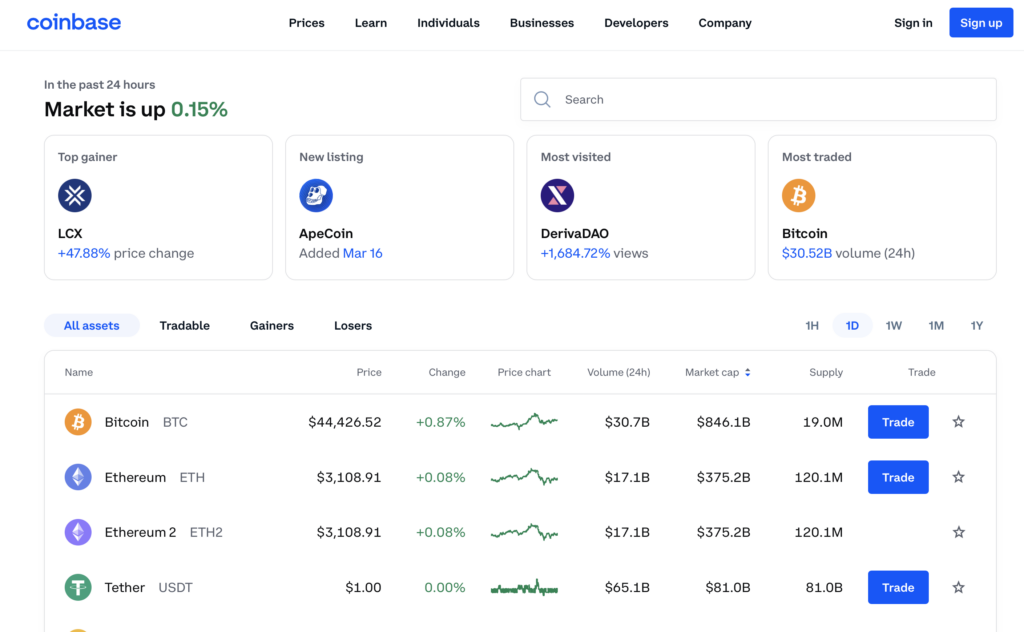The image depicts a detailed Coinbase web page interface. At the top, 'Coinbase' is prominently highlighted in blue. To the right are various menu options in black text, including 'Prices,' 'Learn,' 'Individuals,' 'Businesses,' 'Developers,' and 'Company,' followed by a longer gap and then 'Sign In.' Adjacent to these options is a small blue rectangle with the words 'Sign Up' in white font. 

Below, a summary indicates the market performance over the past 24 hours, stating boldly in green that the market is up by 0.15%. To the right, an empty search bar labeled 'Search' with a magnifying glass icon is visible. 

The page then presents information on 'Top Gainer,' 'New Listing,' 'Most Visited,' and 'Most Traded' assets. Further categorization is provided under labels: 'All Assets,' 'Tradable,' 'Gainers,' and 'Losers.' 

A comprehensive graph is present with columns labeled 'Name,' 'Price,' 'Change,' 'Price Chart,' 'Volume (24H),' 'Market Cap,' and 'Supply,' with up and down arrows for sorting. The final column is 'Trade.' Under the 'Name' column, cryptocurrencies like Bitcoin, Ethereum, Ethereum 2, and Tether are listed, each accompanied by respective numeric values for the other columns.